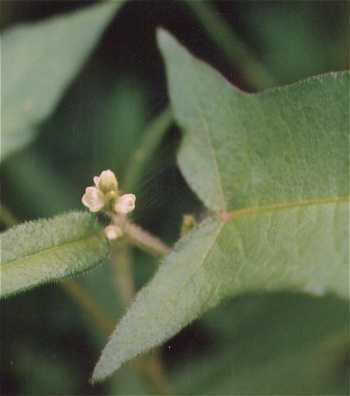This close-up photograph, taken in a nature setting, features a detailed view of a budding flower amid lush greenery. The foreground prominently showcases a leaf on the right-hand side that is rectangular at the base and fans out like a fin towards the center, featuring a lighter green central vein and fuzzy, velvety tips. Protruding from or behind this leaf is a light-colored stem topped with a small bud adorned with four tiny white flowery objects just beginning to blossom. To the left, another smaller oblong and fuzzy leaf is visible. The backdrop, a tapestry of blurred foliage in various shades of green, dark areas, and hints of brown, subtly fades into the background, highlighting the intricate details of the budding flower. This image captures the intimate beauty of nature's delicate growth.